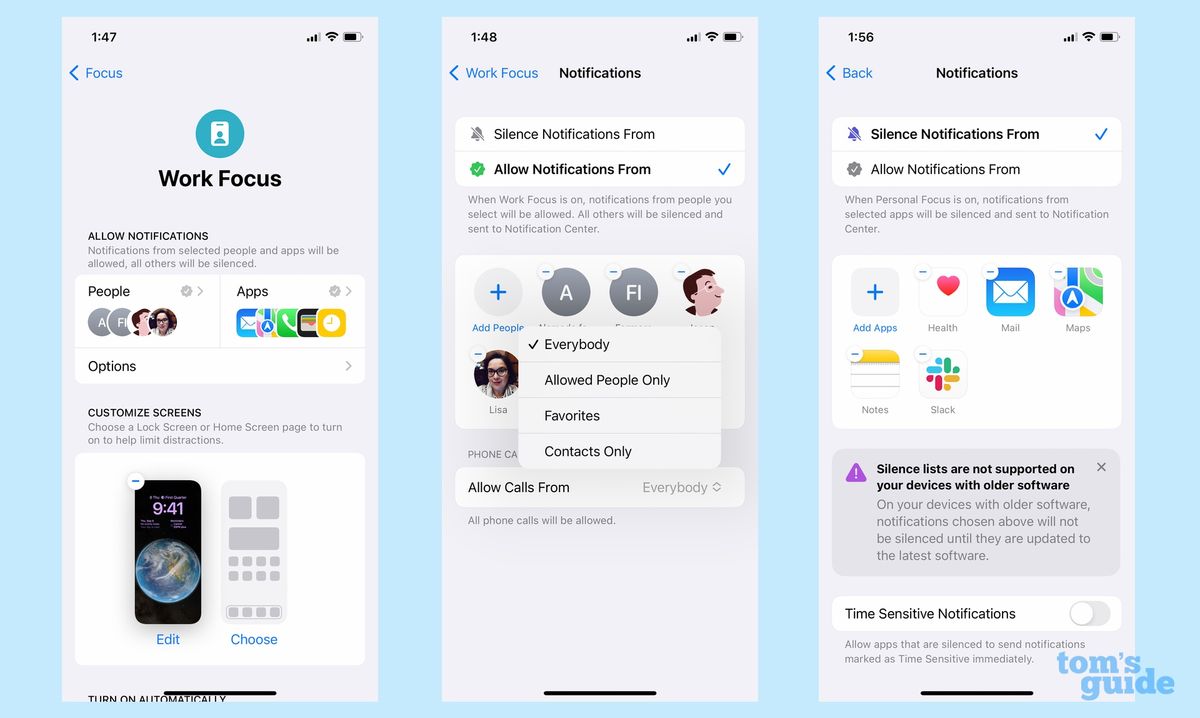The image features a light powder blue background with three evenly spaced panels, each with a light gray backdrop. 

**Left Panel:**
- At the top, the text '147' is displayed.
- Icons for cellular signal strength, Wi-Fi, and battery status are situated on the right.
- Below this, a blue arrow pointing left is labeled 'Focus'.
- In the center of the panel, a turquoise blue circular icon contains the initials 'WF' for 'Work Focus' displayed underneath.
- Text reads 'Allow Notifications', followed by listing options for 'People', 'Apps', and 'Options'.
- There is a visual representation of a cell phone alongside 'Customize Screen', and options to 'Edit' and 'Choose'.

**Center Panel:**
- The top displays '140' with the same signal, Wi-Fi, and battery icons on the right.
- The text 'Work Focus' appears in blue.
- The central text reads 'Silence Notifications From' and 'Allow Notifications From', with the latter ticked off.
- Several circles act as icons for 'Add People', followed by a plus sign, and initials 'A' and 'FI' alongside a cartoonish person image.
- A person named 'Lisa' appears among allowed people, with options to filter notifications to 'Favorites' and 'Contacts Only' or 'Everybody'.
- The panel notes 'Allow Calls From Everybody' at the bottom.

**Right Panel:**
- At the top, '156' is displayed with the same set of icons on the right-hand side.
- A back arrow labeled 'Back' is at the top followed by 'Notifications' in the center.
- Below, texts read 'Silence Notifications From' and 'Allow Notifications From', with a checkmark beside the latter.
- A list of different apps follows, including 'Health', 'Mail', 'Maps', 'Notes', and 'Slack'.

Each panel collectively illustrates different aspects of managing notifications and setting preferences for a 'Work Focus' mode.